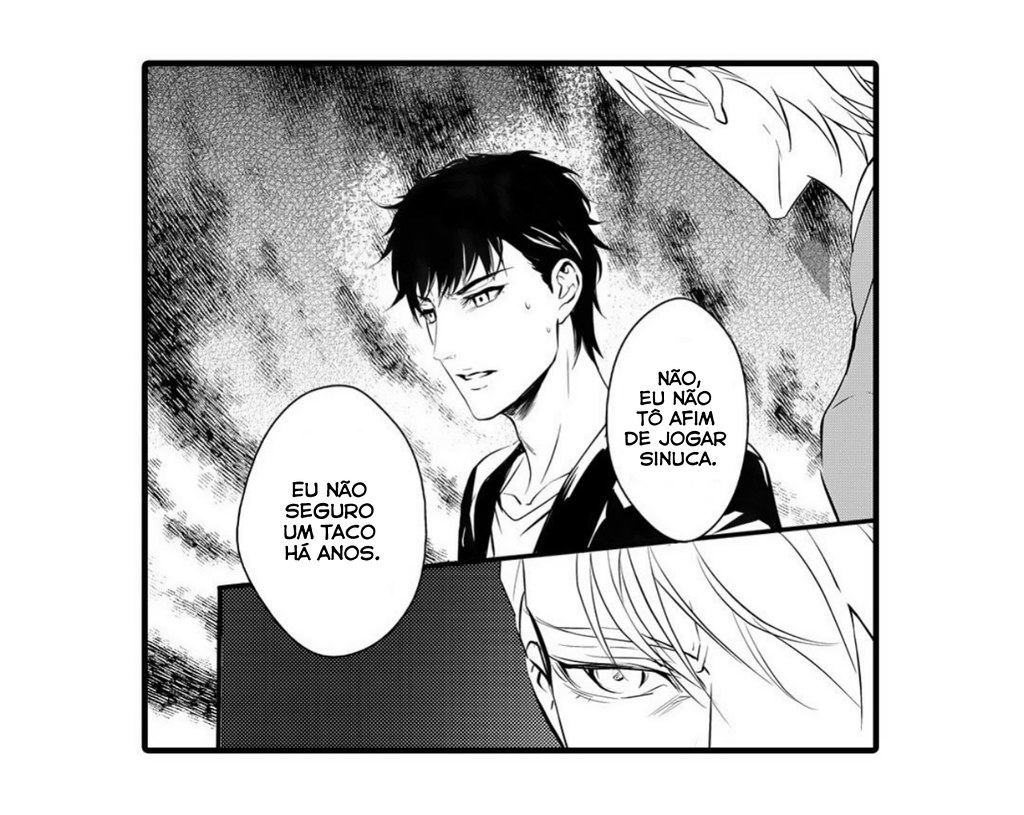The image depicts a black and white square comic book panel featuring two male characters engaged in a serious conversation in what appears to be Spanish. The panel has a distinct cartoonish nature with detailed shading in dark gray, light gray, white, and black.

In the upper section of the panel, the central character, a boy with spiky black hair and white highlights, is prominently featured. He is looking towards the left side of the image and is dressed in a black jacket. Next to him, a friend with blonde hair is partially visible, primarily from his chin and side of the face.

The bottom right portion of the panel zooms in on the face of the second friend, showing just his eyes and the top of his head. Their dialogue, spread across two circular text bubbles in the panel, reads: "inau seguro em tako ha anos" and "nau eo nau ta afem de joga senuka." These exchanges hint at a somber or serious topic being discussed between the characters.